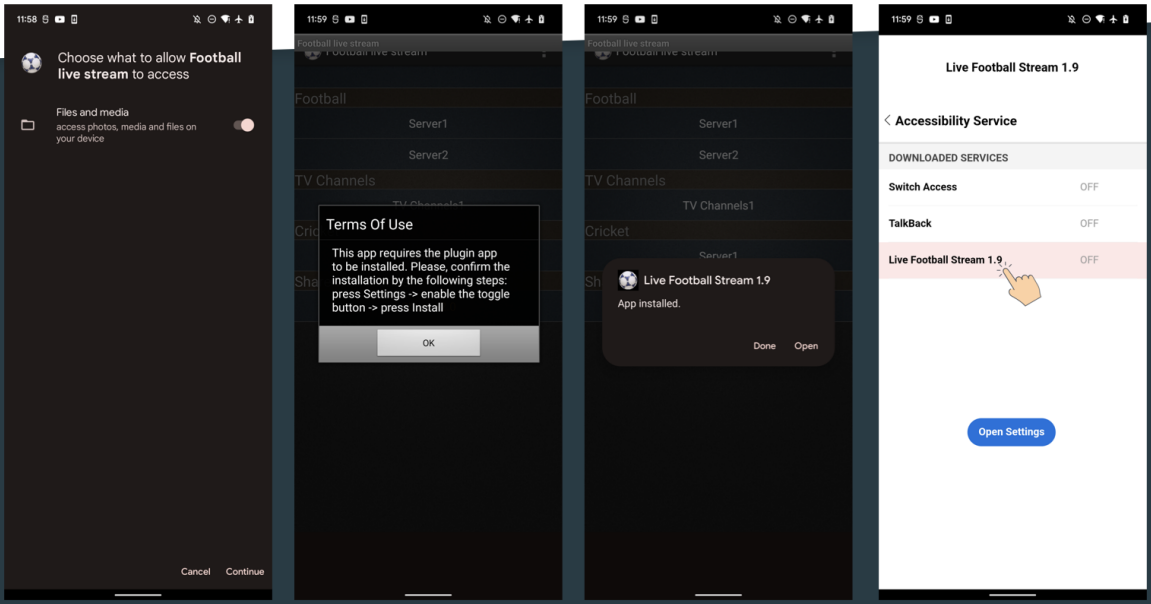The image is divided into four separate screenshots, each displaying different stages of setting up a football livestream app on a smartphone.

1. **First Screenshot (Far Left):** The app interface has a black background and displays a permission request. At the top, it reads "Choose what to allow Football Livestream to access." Below this, there's an icon representing football in white and navy. A highlighted option labeled "Files and media: Access photos, media, and files on your device" is turned on, indicated by a pink toggle switch.

2. **Second Screenshot (Second from Left):** This central image shows a pop-up notification with the title "Terms of Use." The notification, set against a black background with white text, informs the user that the app requires a plugin to be installed. It provides the following instructions: "Please confirm the installation by following the steps: Press Settings, enable the toggle button, tap Install." At the very bottom, there is a grey "OK" button. Partially visible behind the pop-up are texts like "Football Livestream" and "TV channels," but these are mostly obscured.

3. **Third Screenshot (Second from Right):** This image repeats the black background with partially obscured text seen in the second screenshot. However, the new pop-up reads "Live Football Stream 1.9 App installed" and presents two buttons at the bottom: "Done" and "Open."

4. **Fourth Screenshot (Far Right):** The final image shows a white background detailing the accessibility service settings for the "Live Football Stream 1.9" app. The section lists several services: "Switch Access" (off), "TalkBack" (off), and "Live Football Stream 1.9" (off), alongside an instructional hand icon to activate the service. A blue "Open Settings" button is located at the bottom.

This detailed caption specifies each step and visual element involved in setting up the app, ensuring clarity and thoroughness.